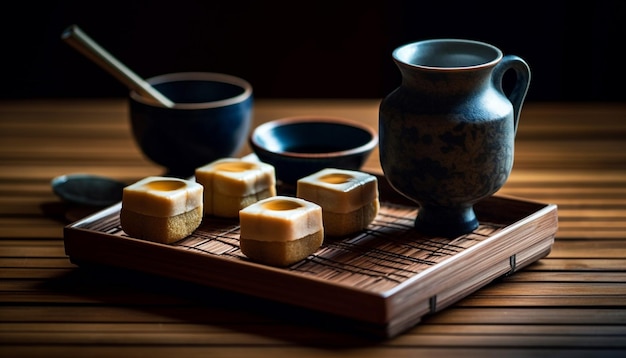This atmospheric image portrays an intricate matcha tea ceremony setup on a wooden bamboo table. Central to the scene is a small, rectangular, light bamboo serving tray with a visible wireframe structure, aiding its integrity and portability. The tray contains several handcrafted, marble-esque ceramic items, all in earthy, dark hues.

To the upper right of the tray is a dark blue, oval-shaped teacup with a delicate handle. Adjacent to this, sits a small brown bowl. Four distinct tan to orange cubes with circular hollows occupy the front left corner of the tray, reminiscent of artistic erasers or miniature baskets. 

In the background to the left, a black matcha bowl accompanied by a white stirring stick rests thoughtfully, suggesting meticulous preparation. On the table's left side, outside the tray, another small serving cup or possibly a bowl can be seen, hinting at additional traditional utensils for the ceremony.

The entire arrangement is highlighted against the rich tones of the bamboo wood table, exuding an aura of cultural precision and ceremonial artistry, captivating the moody, intimate lighting of the photograph.